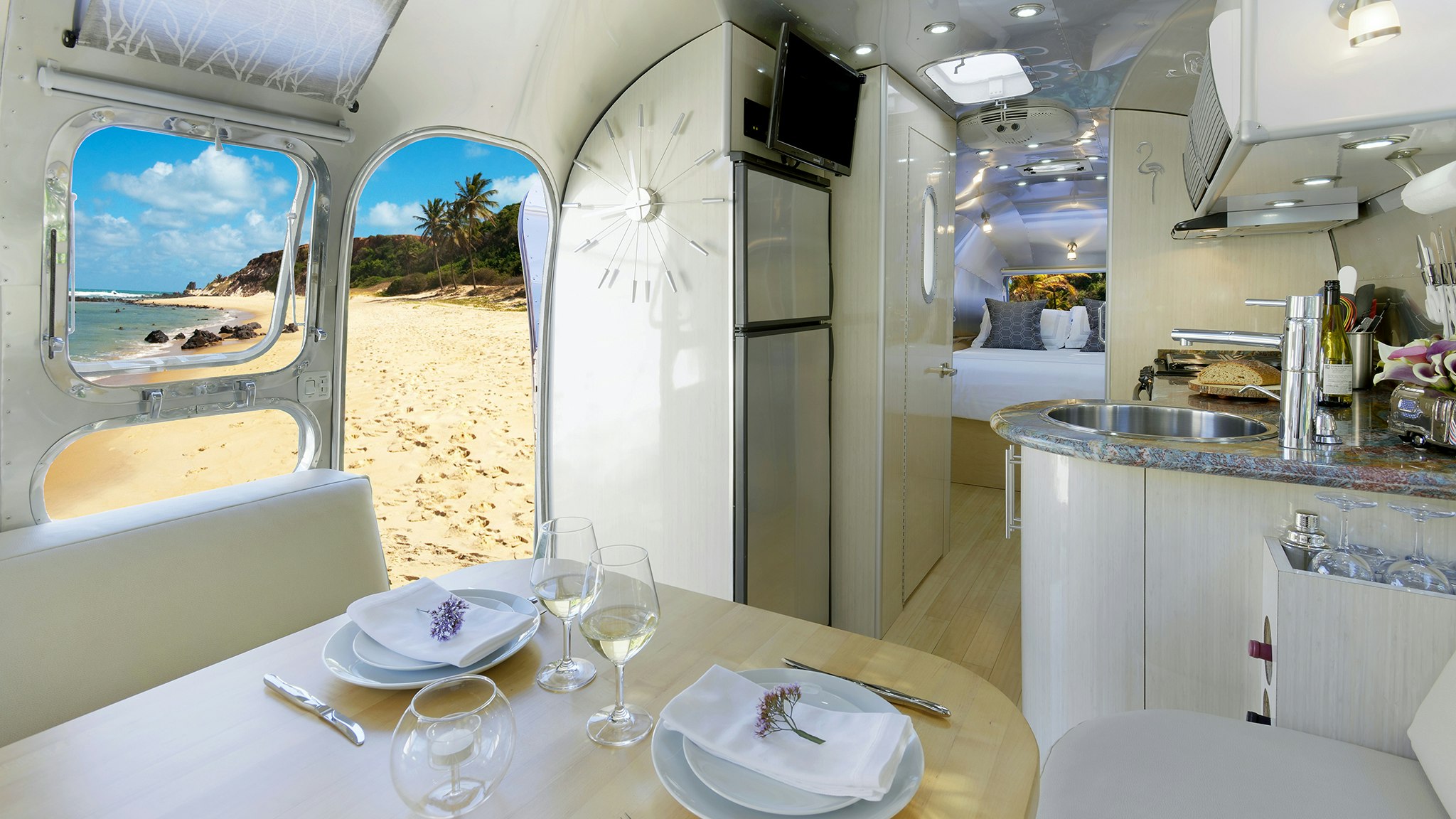The image portrays the interior of a modern RV camper, possibly an Airstream, with a retro-modern design. The camper's interior is predominantly white with beige accents. Central to the image is a light-colored wooden table, set for four with white plates, silverware, and two glasses containing a tan liquid, possibly champagne. Two white bench seats flank the table, each adorned with a napkin and a small flower.

To the left of the table, there's a large window and an open door that leads to a beach. Outside, tan sand, clear skies with clouds, blue ocean water, and palm trees create a serene backdrop. A pair of hills are visible in the distance.

On the right side of the image, the RV features a stylish kitchen area with gray countertops and stainless steel appliances, including a sink. Adjacent to the kitchen area, a silver-colored refrigerator is built into the wall, topped with a small TV. Above the refrigerator, a starburst clock adds a vintage touch to the decor.

Further back, down a hallway, there is a bedroom area with a neatly made white bed covered with multiple pillows. The overall design is cohesive, blending modern amenities with a nostalgic flair, all set against a picturesque seaside view.